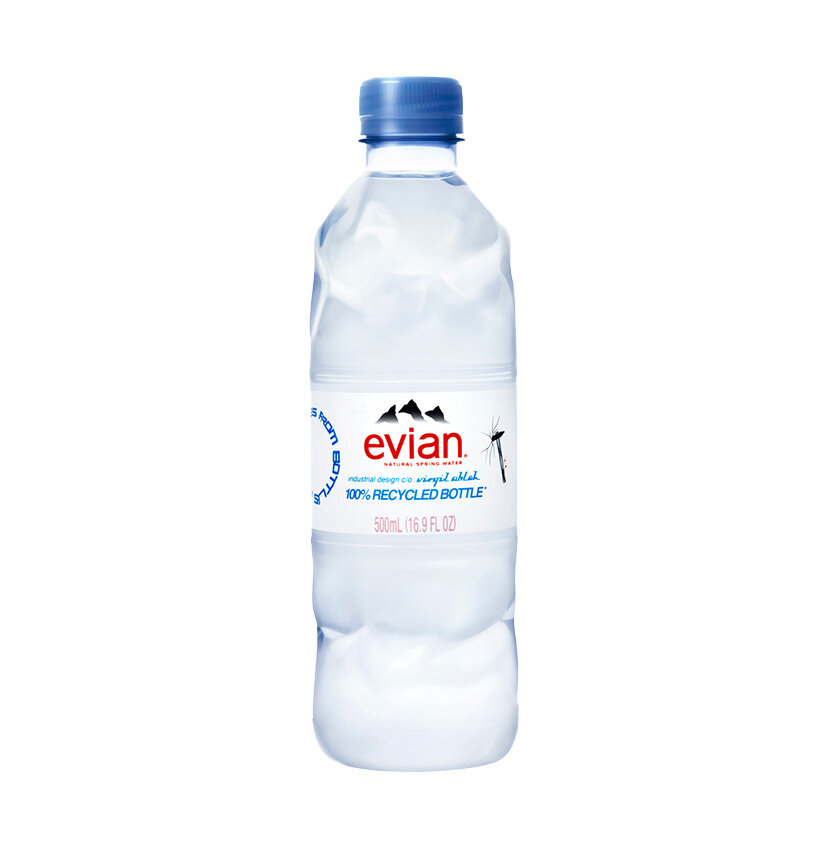The image depicts a bottle of Evian natural spring water. The bottle is clear with a slightly crinkled appearance and features a blue cap. The white label, adorned with a logo of three dark blue mountain peaks, prominently displays the brand name "Evian" in all lowercase, red letters. Below the brand name, "natural spring water" is written, followed by another line in blue text that reads "100% recycled bottle." The label also lists the bottle's capacity, which is 500 milliliters or 16.9 fluid ounces, in a lighter shade of red. The bottle appears to be full and unopened, making it a thirst-quenching sight.